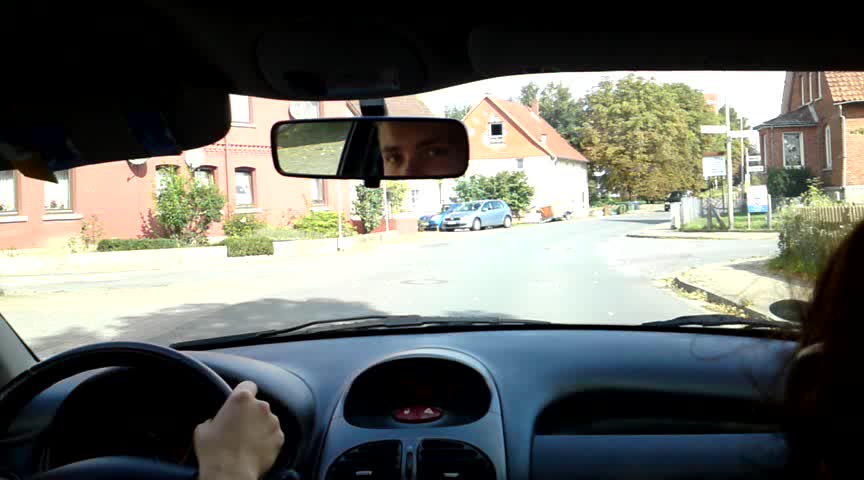A photograph captures an intimate moment inside a car on a bright, sunny day. The image, taken from the backseat, presents a detailed view of the car's dark blue interior. The driver's hand, with light skin, grips the steering wheel, partially visible on the left side of the frame. The driver’s face, from the nose to the forehead, can be seen in the rearview mirror, their gaze directed towards the camera. 

Outside, the scene is bathed in sunlight, illuminating a serene residential area with numerous red brick buildings. Green trees and bushes add a touch of nature to the urban setting. A few blue cars are parked in the distance, and the light gray roads glisten as they reflect the sunlight. The tan-colored sidewalks border the streets, completing the picturesque suburban landscape.